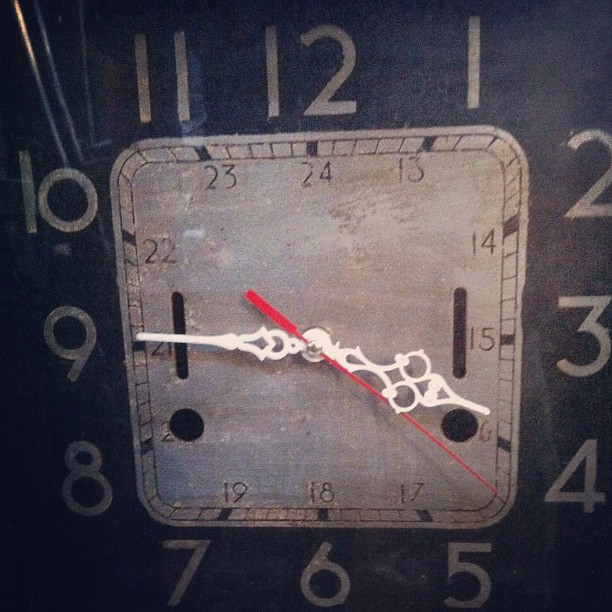This is a close-up photograph of an authentically vintage analog clock dial, capturing the intricate details and wear that attest to its age. The surface shows signs of time-worn patina, indicating it's not a modern reproduction. The hour and minute hands are ornate, though slightly warped, and the second hand, which appears bent and weathered, is currently folded underneath the hour hand, suggesting the clock is not operational and in need of repair. The clock features two dials: a 24-hour clock in the center square and a 12-hour clock on the outer perimeter. Notably, there are keyholes for winding located near the 4 o'clock and 8 o'clock positions, hinting at the internal spring mechanism typical of such vintage timepieces.